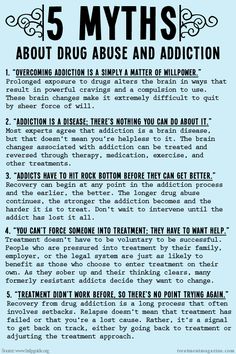The image is an infographic with a blue background and black text titled "Five Myths about Drug Use and Addiction." At the top, there are some designs enhancing the visual appeal. The infographic debunks five common myths, each followed by a detailed paragraph of explanation:

1. **Overcoming addiction is simply a matter of willpower**: It explains that prolonged exposure to drugs alters the brain, creating powerful cravings and a compulsion to use, making it extremely difficult to quit through sheer willpower alone.
  
2. **Addiction is a disease; there's nothing you can do about it**.

3. **Addicts have to hit rock bottom before they can get better**.

4. **You can't force someone into treatment; they have to want help**.

5. **Treatment didn't work before, so there's no point in trying again**.

Each of these myths is accompanied by short paragraphs that elaborate on why these beliefs are incorrect, aiming to provide a clearer understanding of drug addiction and treatment. The layout is well-designed with a pleasant color scheme and an easy-to-read font, making the information both accessible and engaging.